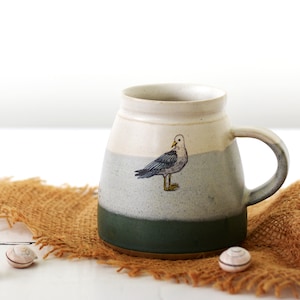This photograph showcases a blue and white stoneware mug that narrows toward the top like a spill-proof travel mug but is crafted from stoneware. The mug features a layered glaze with a top band of white, a broad middle band of light blue that extends onto the handle, and a teal green base. The handle is positioned on the right side of the mug in the photograph. A prominent design element is the seagull decoration; the bird is depicted standing and looking back over its wings. The seagull motif is reminiscent of Japanese Otagiri pottery designs. The mug rests on a loosely woven burlap cloth, with a couple of small snail shells placed next to it. The background is a hazy blue, contributing to the serene, coastal aesthetic of the scene. The setting is indoors, well-lit by natural light, and offers a detailed view of the mug's unique design, color transitions, and accompanying elements.